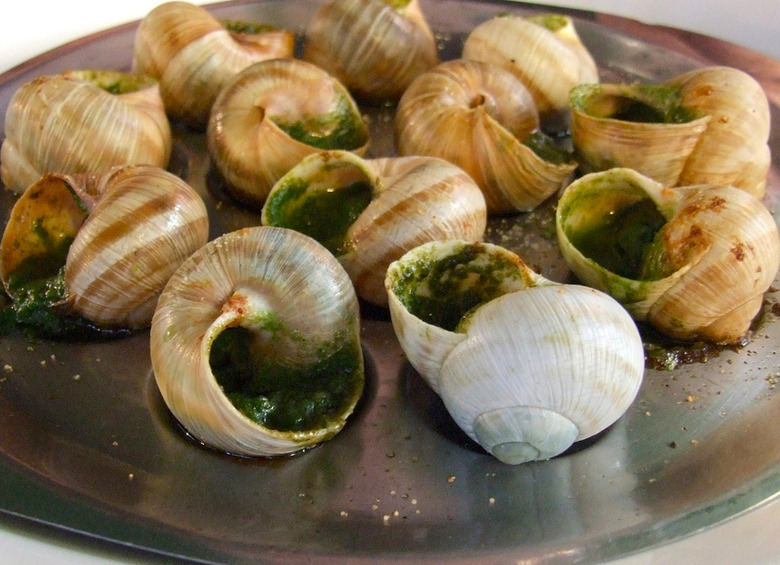This is a detailed close-up, horizontally aligned image of a dish containing roughly 12 escargots. The escargots are arranged on a large round plate with a silvery-greenish and brown-gray hue, possibly metal. The plate sits on a white table, with its edges cut off slightly in the photograph. The foreground features a crisply focused view of the escargots, revealing their brown shells with darker brown stripes. In the center of the plate is a unique white shell, appearing more like an onion with its top part removed, allowing a clear view of the green sauce—likely a pesto or a smashed broccoli mixture—inside the shell. The background escargots appear slightly blurred, adding depth to the image. The plate itself is sprinkled with seasoning, potentially pepper, represented by small dots and crumbs, adding texture to the composition.